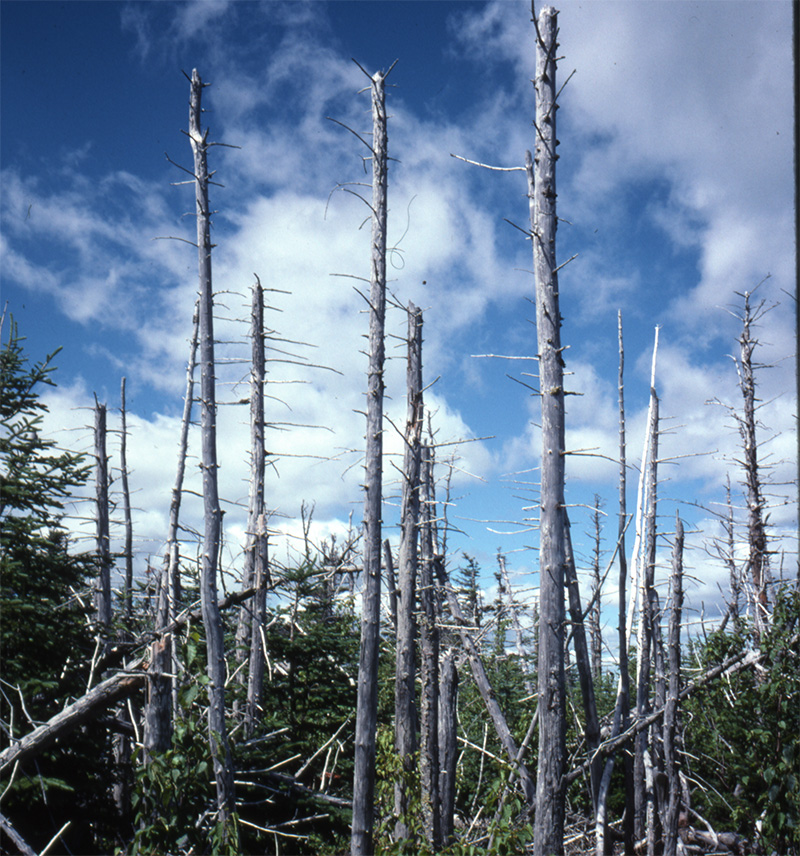The photograph shows a stark contrast between a barren section of what appears to be a forest and the more lush surroundings. Dominating the foreground are tall, gray, thorny plants with long, hard, woody stems, entirely devoid of leaves. These plants, characterized by their fibrous pines, evoke a harsh, arid atmosphere, suggestive of a region that may have endured a traumatic event such as a forest fire, leaving behind only desolate, leafless branches. In vivid contrast, the background and surrounding areas display more vibrant and leafy greenery. Above, the sky stretches out, occupying nearly three-quarters of the image with its serene blue expanse dotted by fluffy white clouds. The scene, bathed in sunlight, emphasizes the juxtaposition between life and desolation in this outdoor setting.